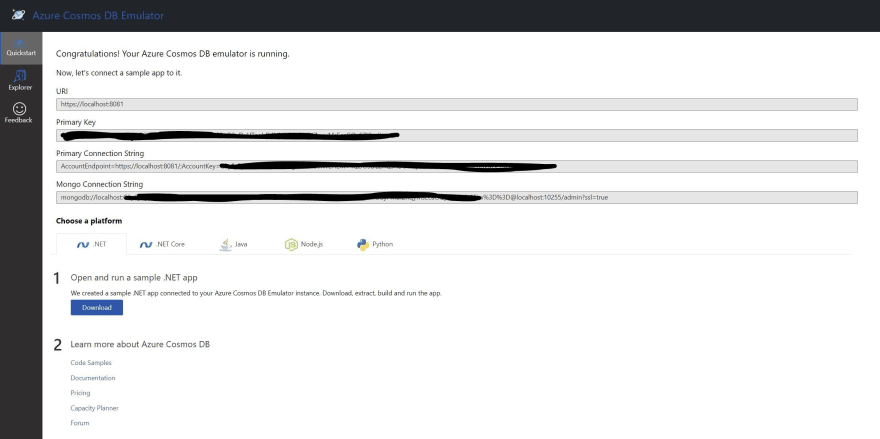The image depicts a screenshot of a web page that appears to contain classified documents. The page includes several text boxes, some filled with text, while three of these boxes are redacted with thick black lines, concealing their contents. Within the layout, approximately halfway down on the left-hand side, there is a distinct blue box. This blue box is framed at the top with a black border, making it stand out from the rest of the page. The overall composition suggests restricted and sensitive information, highlighted by the prominent redactions.